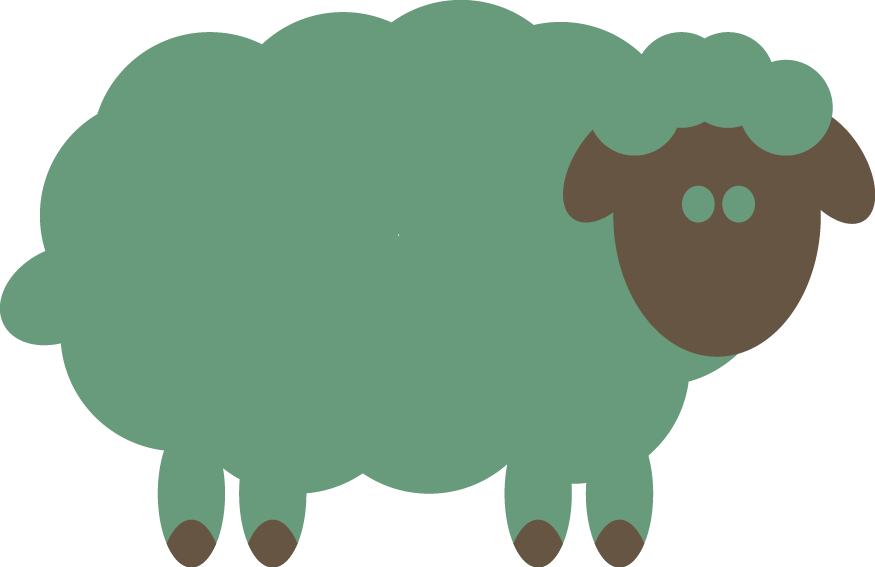This is a simple yet stylistic depiction of a big green sheep, likely created with a digital program. The sheep's body resembles a puffy cloud and is uniformly green. Its fur has the appearance of a flat, solid color without texture, and it sports a short, stubby tail of the same green hue. The face and feet are brown, with the feet depicted as small brown spots at the end of four stubby, straight legs. The face has two green circles for eyes, but no visible nose or mouth. The image captures the sheep looking straight ahead, and its overall simplicity suggests it could have been made with basic digital art tools, though the quality is notably higher than that typically associated with basic software like PowerPoint.